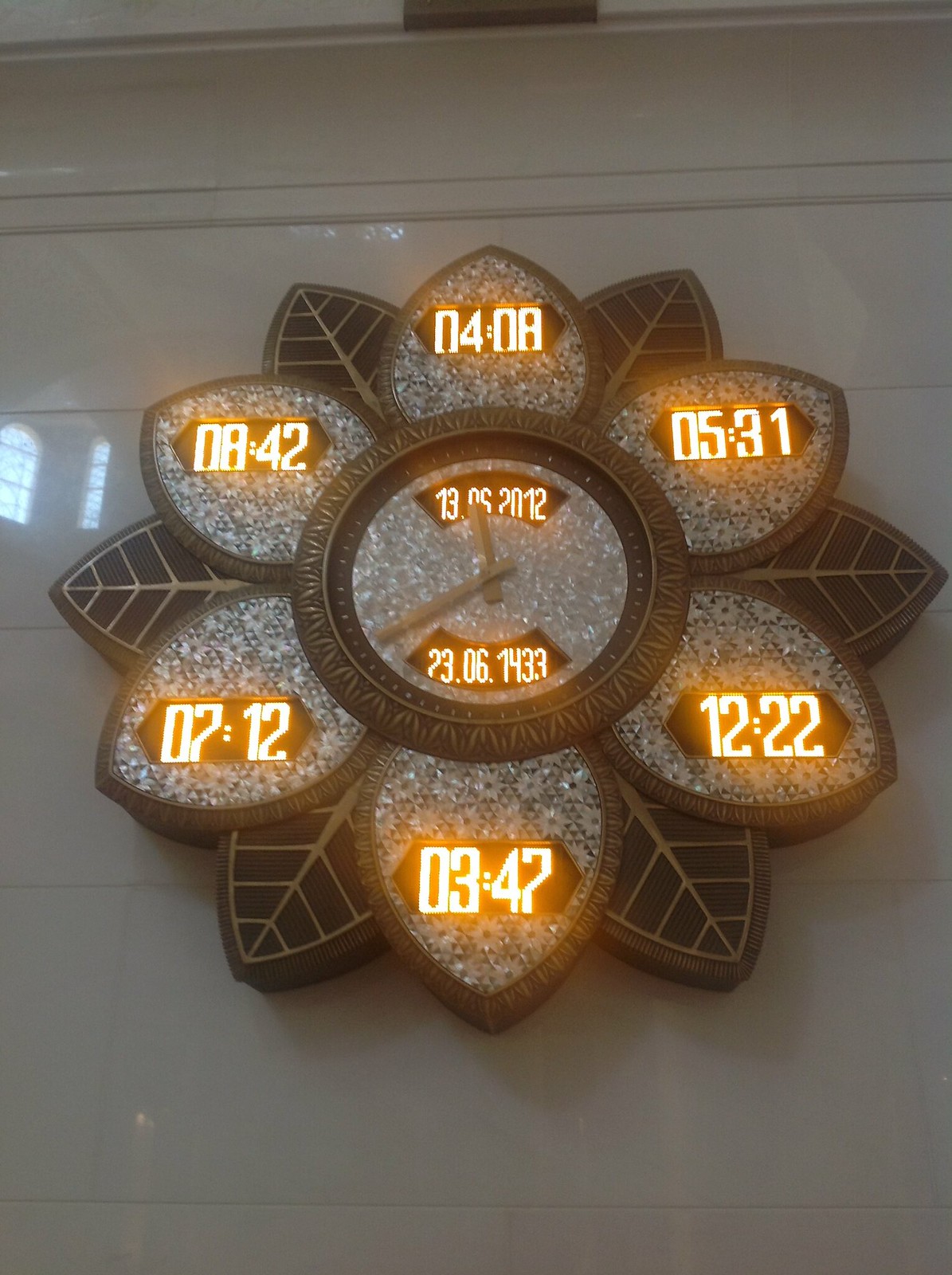This is an image of a uniquely designed clock that resembles a flower. The clock features six petal-like sections, each displaying different numeric values in orange-colored digital lettering. The petal at the top displays "408," the petal to the top right shows "0531," followed by the petal on the right with "1222." The petal at the bottom reads "0347," moving to the lower left it shows "0712," and the upper left petal displays "0842." 

In the center of this floral clock, there is a traditional analog clock face with hour and minute hands. The time on the analog clock reads "13:00" or a short moment past the hour, obscured by the hour hand. Within this central area, additional digital times are displayed: at the top, it reads "2012," in the middle "2306," and at the bottom "1433." 

The intricate design combines both analog and digital elements to create a visually striking and complex representation of time.